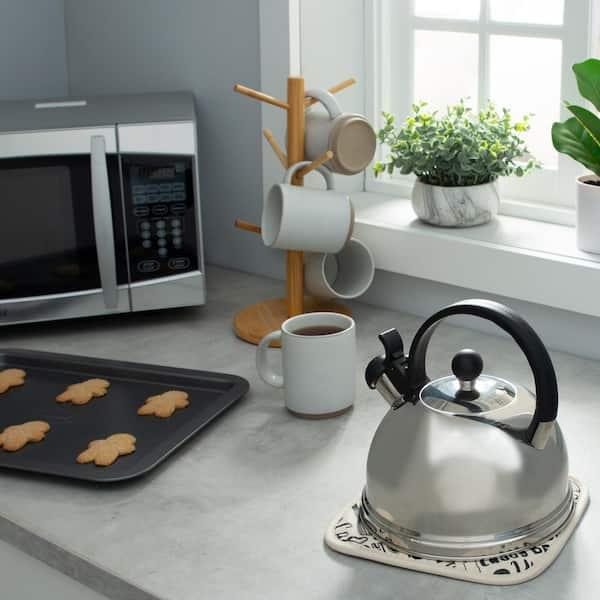The image depicts a modern kitchen scene, thoughtfully arranged to highlight a balance between function and aesthetic appeal. At the center of the gray countertop, there resides a silver teapot with a sleek black handle, placed meticulously on a rounded square tray adorned in white and black hues. Adjacent to this, positioned slightly above and to the left, is a pristine white mug containing a dark liquid, likely tea or coffee. Behind the teapot setup stands a charming wooden stand designed like a miniature tree, elegantly displaying three additional white mugs. On the right side of the stand, a windowsill painted in crisp white hosts a couple of verdant plants, adding a touch of natural greenery to the composition. To the left of the mug stand, a silver microwave with black accents integrates seamlessly into the kitchen decor. Completing this cozy and inviting scene, a metal cookie sheet laden with perfectly baked gingerbread cookies rests on the same gray countertop, indicating a delightful blend of culinary activity and warm, homely atmosphere.